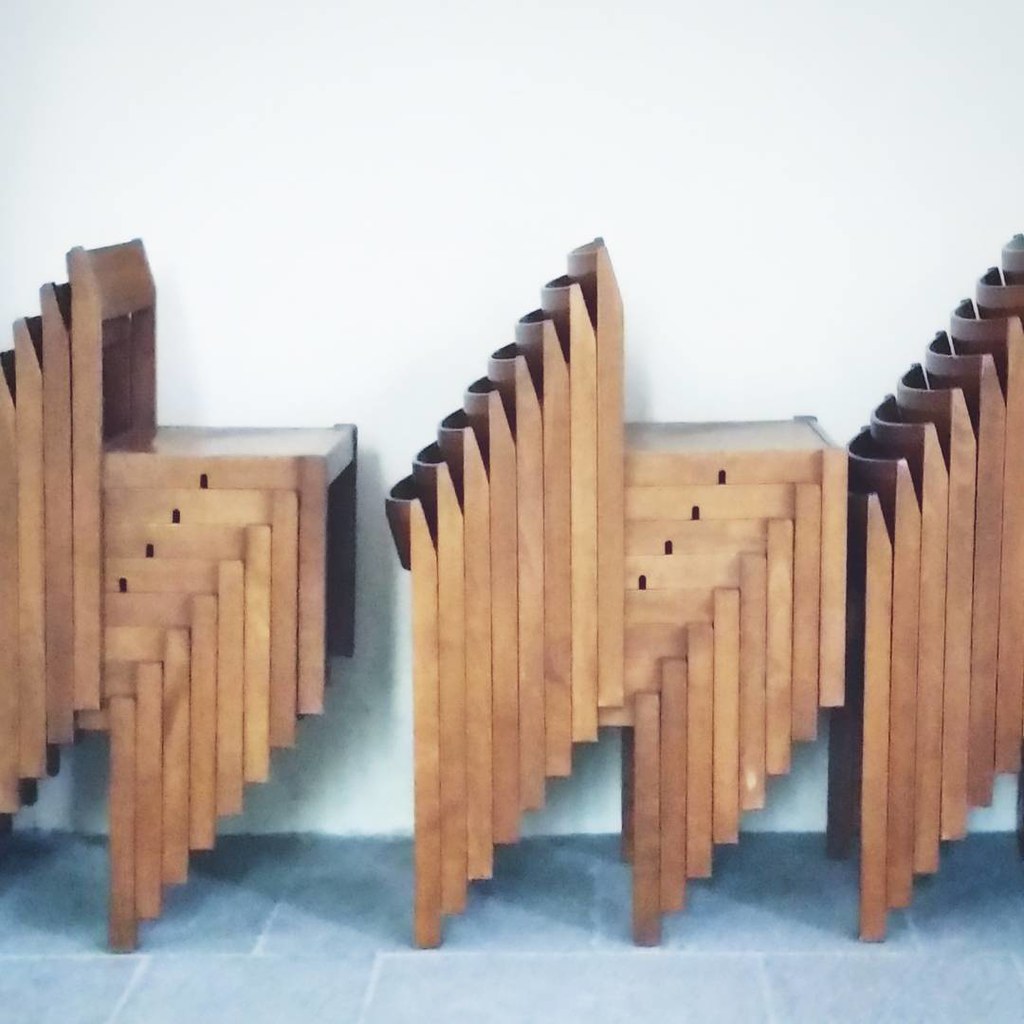The image showcases a room with a gray tiled floor and white walls, where three meticulously arranged stacks of wooden chairs are positioned against the back wall. Each stack consists of approximately eight to nine chairs, all identical and artistically interlocking in a manner that forms a cohesive and orderly pattern. The vertical backs, front legs, and seats of the chairs align perfectly, creating the illusion of two standing parallelograms flanking a central cube. The middle stack is fully visible, while the stacks to the left and right are partially cut off by the frame, revealing only the vertical lines of the chairs' backs. The chairs all face the same direction, with their seats pointing to the right, contributing to the geometric harmony and aesthetically pleasing composition of the scene.